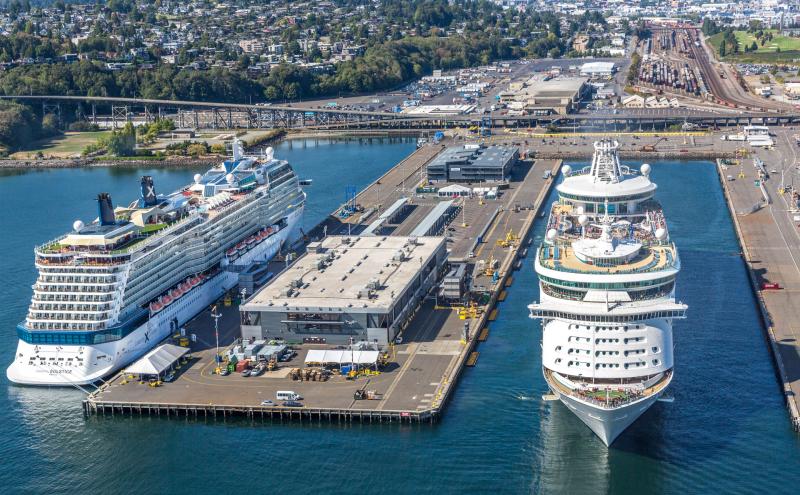The photograph captures a detailed scene of two enormous cruise ships docked at a bustling harbor. The image, taken from a high vantage point—likely a tall building—looks down onto the scene. The foreground is dominated by the striking presence of two colossal, white luxury liners: the ship on the left is docked and facing away, while the one on the right is making its way into the port, facing the camera. The sheer size of these multi-storied vessels is emphasized by the bustling activity around them, with people standing on the decks, observing the docking process.

The harbor itself is a well-constructed area made of cement, surrounding the ships with buildings centrally located on the dock. This rectangular platform in the middle of the water includes white and grey warehouses; the white one possibly used for boarding luggage, and the smaller grey warehouse approximately 100 yards away. Additionally, there are two tents used for storing vehicles. Overhead, a bridge or overpass connects to the harbor, underscoring the port's integration into the urban landscape.

In the background, the upper third of the photo showcases a cityscape abundant with trees on the left and an industrial area with large stacked containers on the right. A sprawling outdoor parking lot filled with cars adds to the sense of scale and activity. The overall scene is bathed in daylight, providing a clear and vibrant snapshot of the port's dynamic operations.